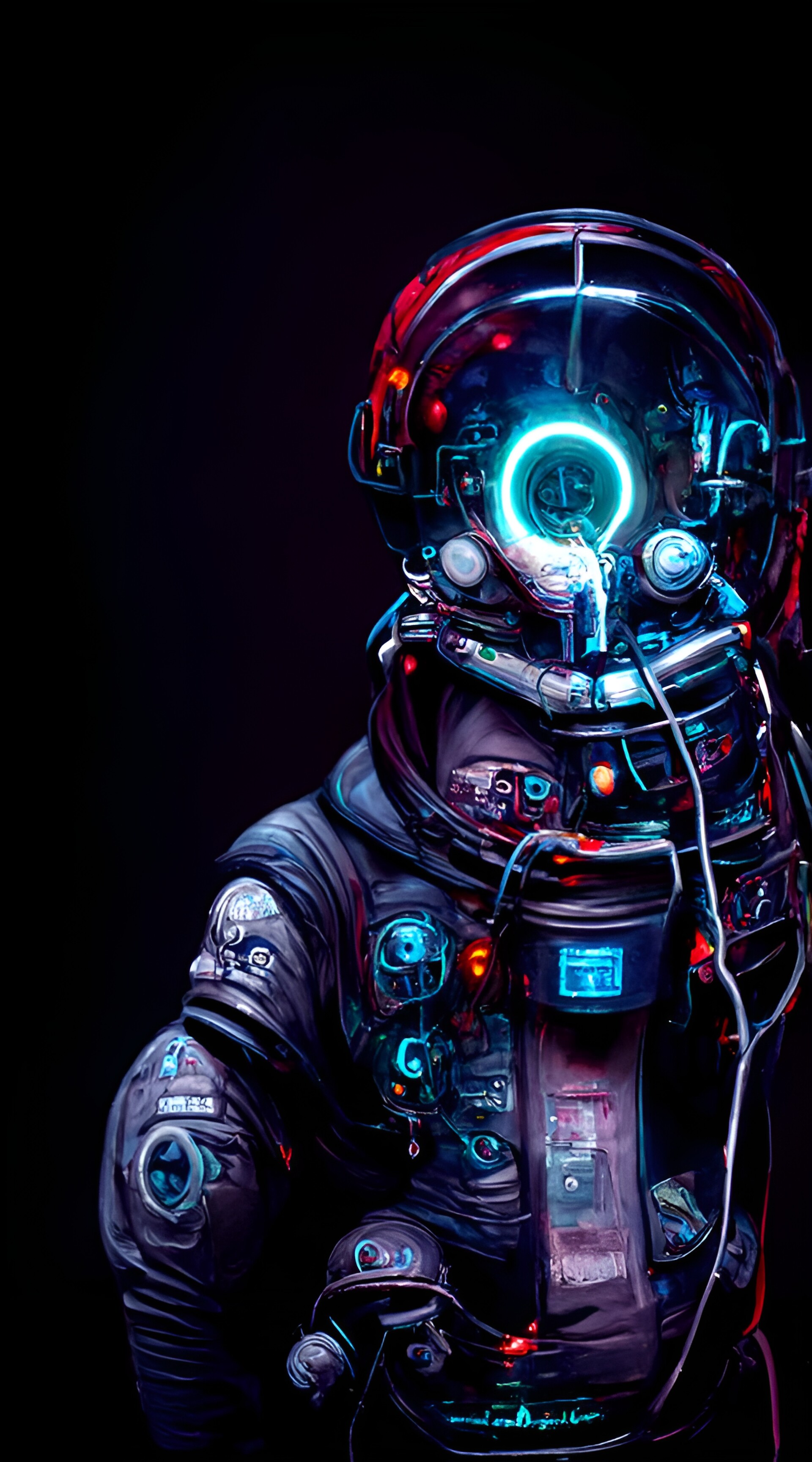The image showcases a robot-like astronaut suit, primarily highlighted by a dark purple exterior with light blue illuminated accents. The suit has intricate dark blue detailing and various buttons and gears on the right arm and front torso. Although only depicted from the waist up, additional elements include white tubes emerging from the left side of the helmet and merging into a single tube extending towards the bottom left of the image. The helmet, semi-transparent and glass-like, reveals an array of gadgets and devices inside, giving it a sophisticated appearance. Notably, where the face should be, there is a glowing blue light, resembling a light bulb. The entire figure is positioned on the right side of a vertically framed black background, partially cut off, emphasizing the suit's front and right arm, but omitting any view of the left arm or hands. The image conveys a futuristic, almost otherworldly atmosphere with its blend of modern and classic astronaut design elements underlined by a mix of light and dark hues.